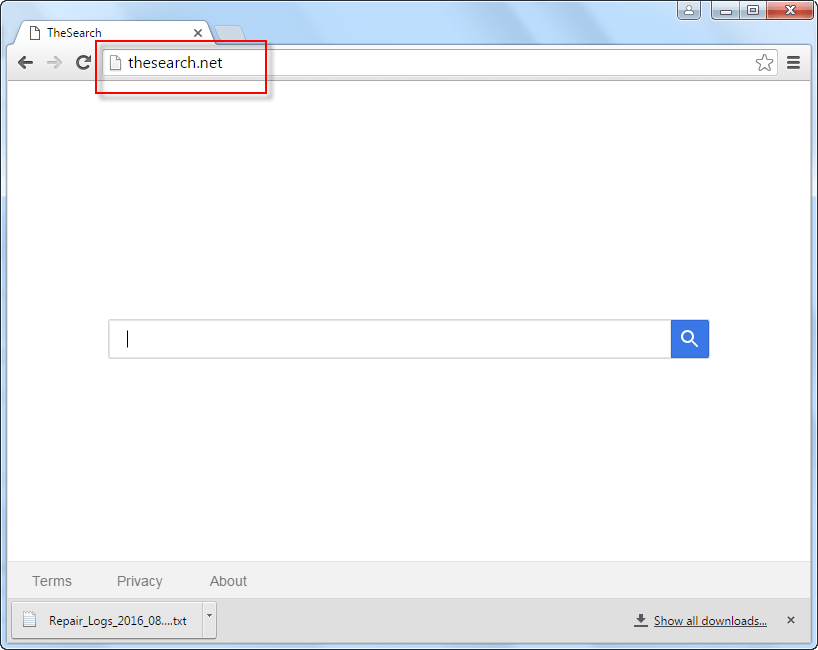This image depicts a website titled "The Search." The top of the website is marked by a light blue bar, which contrasts with the black background that represents the entire computer interface. Below this bar, a white rectangular space dominates the screen. In the browser's address bar, the URL "thesearch.net" is typed in and highlighted in red. Centered on the page is a search bar with nothing typed in it, only the blinking cursor is visible on the left side.

Directly beneath the search bar, a light gray menu contains the options "Terms," "Privacy," and "About." Below this menu, a darker gray box displays a file name: "repair_logs_216_08....txt." Adjacent to this file name, a small download icon is visible with the label "Show all downloads" underlined in black. To the far right of this label, there is a very small X icon located in the lower corner of the screen.